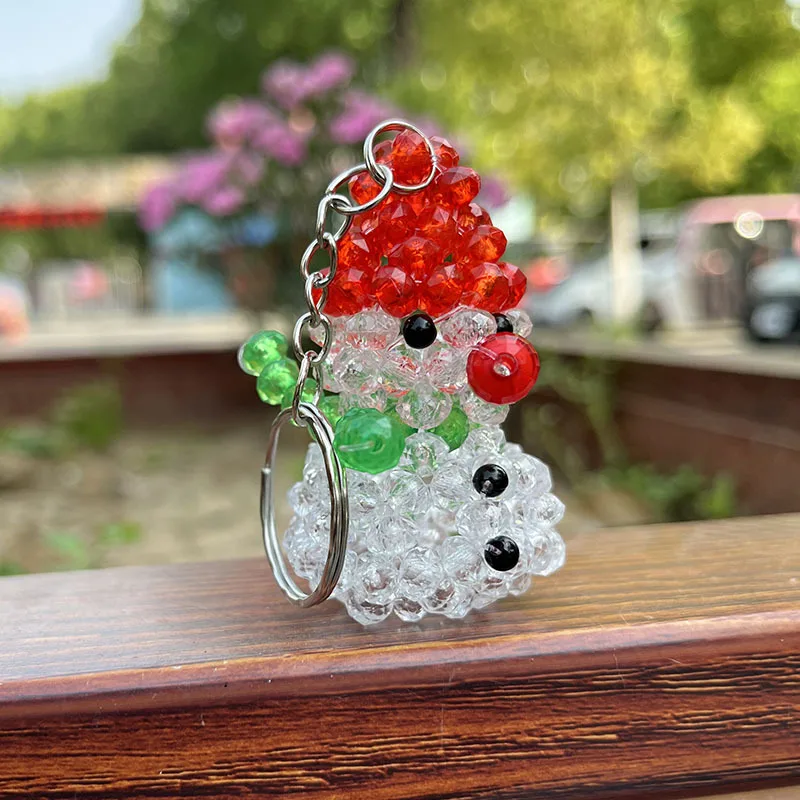This close-up image showcases a meticulously crafted keychain in the shape of a snowman, composed entirely of small, colorful beads. The snowman's body is made from white beads, accentuated by black beads for its eyes and buttons. A striking red bead forms its nose, while a cluster of smaller red beads fashion its cozy hat. A string of green beads intricately creates the appearance of a scarf, seemingly blowing in the wind to the right, adding a dynamic touch to the static figure. At the top of the snowman, a metal keychain loop is attached by a small chain, ready for use. The keychain is positioned on a dark red wooden railing, gleaming with subtle highlights.

In the background, everything is beautifully out of focus, adding depth to the scene. You can discern elements of an outdoor setting, including pink flowers in what appears to be a large planter, various plants, and a tree. Sunlight reflects off the windows of a vehicle further back, adding a touch of sparkle. The sky peeks through a corner, revealing a clear blue hue. Off to the back left, there is a hint of what might be a gas station, completing the picturesque outdoor tableau.